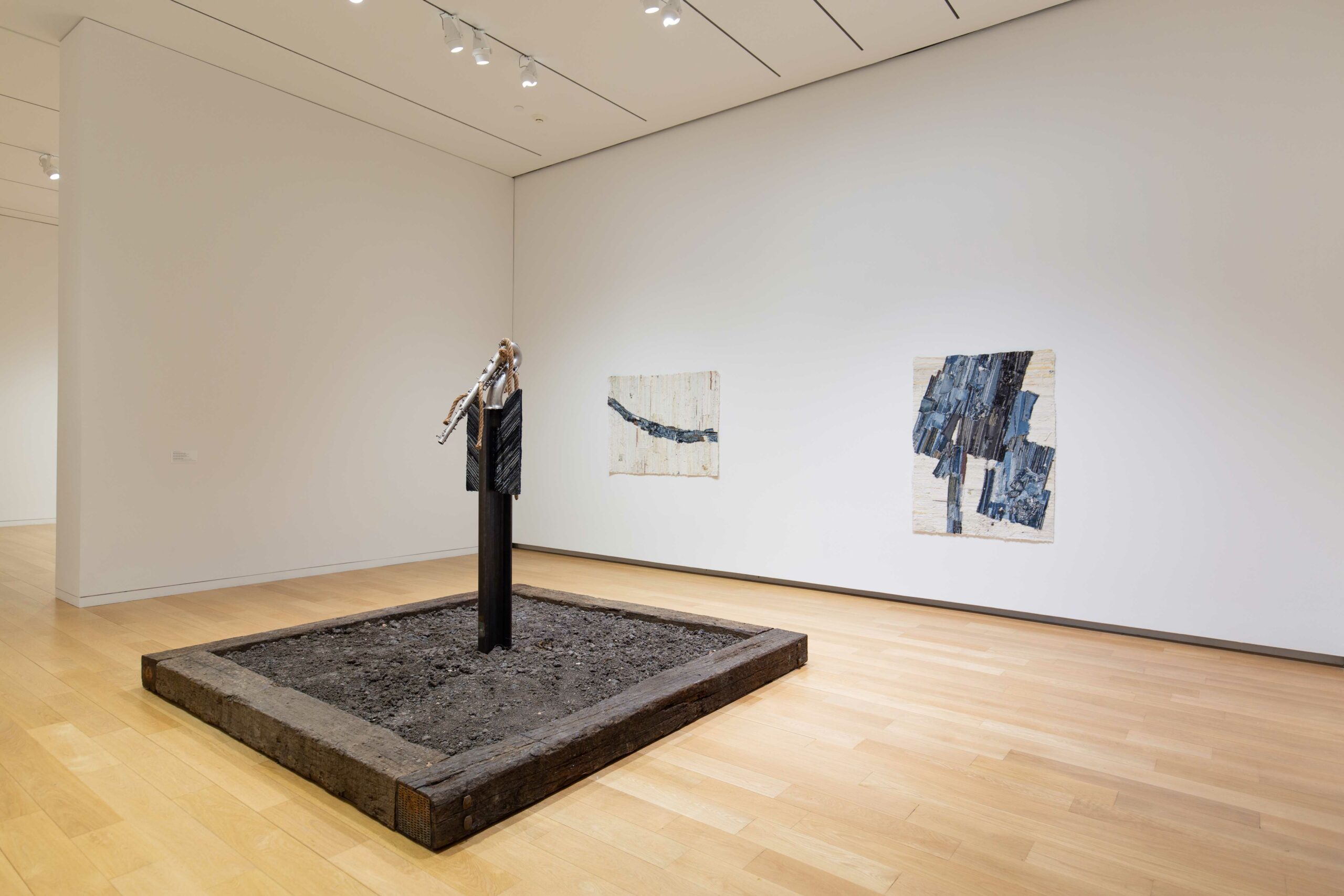This image captures the interior of a modern art gallery with stark white walls and a light hardwood floor. The room features an intriguing central installation, comprised of large wooden beams forming a square base filled with dark soil or gravel. Rising from the center of this base is a thick vertical post adorned with a silver, S-shaped handle wrapped with a piece of rope, which vaguely resembles the handle of a water pump or a brass instrument like a saxophone, pointing downwards.

Two large abstract paintings adorn the converging white walls at the back of the room. The left painting features vivid squares and rectangles in shades of blue, dark blue, and purple set against the white backdrop. The right painting, utilizing a similar color palette, displays a diagonal rod or line stretching from the upper left to the center right of the frame. Both pieces maintain a minimalist aesthetic with no other discernible elements.

Illuminated by tracks of overhead lights, the setup creates a curious and contemplative atmosphere. A black sign with unreadable white text stands in front of the central installation, adding to the enigmatic nature of the exhibit.